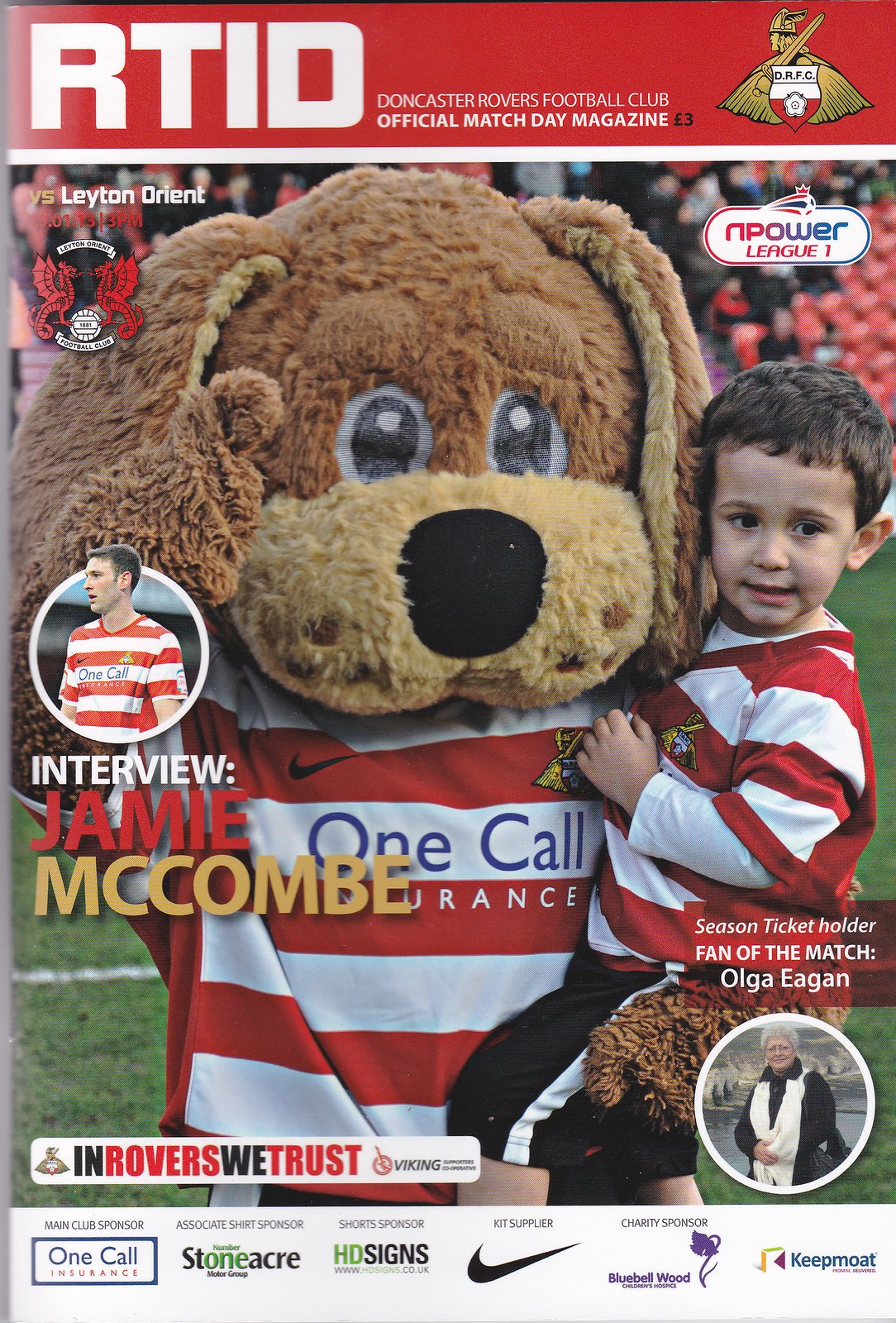The cover of the official match day magazine for the Doncaster Rovers Football Club features a vibrant and engaging design centered on the club's mascot, a brown puppy with floppy ears dressed in a red and white striped shirt, holding a young boy who is similarly attired. The boy's gaze is turned away, adding a bit of candid charm to the scene. Above this main image, against a red banner background, the magazine proudly titles itself "RTID, Doncaster Rovers Football Club, official match day magazine." The top part of the cover also notes that the Rovers are playing Leyton Orient today in the Empower League One, at 3 p.m. on January 19th, 2013. 

To the side, a small round picture features a player named Jamie McComb, highlighted by an article titled "Interview Jamie McComb." Another small round photo in the bottom right corner showcases Olga Egan, recognized as the season ticket holder and fan of the match, with a text header indicating her accolade. At the magazine's bottom, beneath the slogan "In Rovers We Trust," are six sponsor logos, rounding out the cover's detailed presentation. The backdrop hints at a football field, adding context and excitement for the game day featured within.